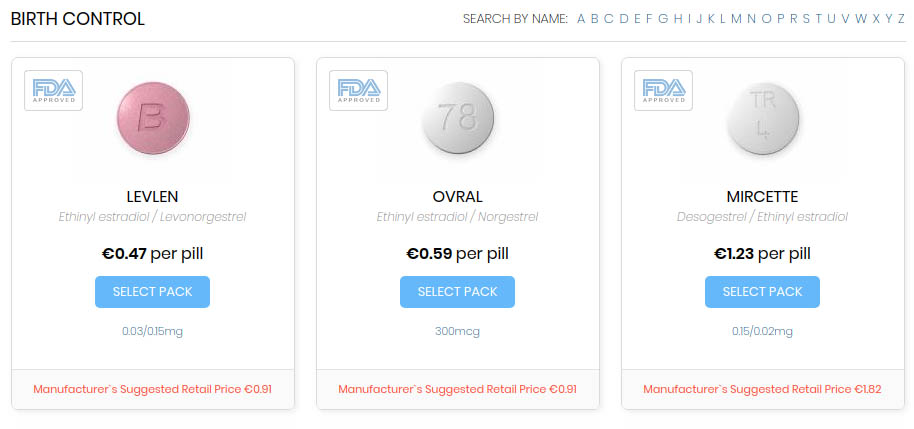In the image, an online pharmacist is presenting a variety of FDA-approved birth control pills. The top left corner prominently displays the heading "BIRTH CONTROL" in bold black letters while the far right features a search function labeled "SEARCH BY NAME" with an alphabetic navigation option from A to Z in blue and grey letters.

The first option presented is a pink pill marked with a "B," which seems to suggest it as a Plan B alternative. The active ingredients listed for this pill are levulin ethanol estradiol and levonorgestrel, a form of progesterone. It is priced at 0.47 euros per pill, with options for 0.03 or 0.15 milligram doses. Below this, the Manufacturer's Suggested Retail Price (MSRP) is noted as 0.91 euros.

The second option is a white pill engraved with "78." The active constituents are ethanol estradiol and norgestrel. It’s priced at 0.59 euros per pill, with dosage options of 300 micrograms. Its MSRP is also 0.91 euros.

The final option displayed is a pill engraved with "TRL." The ingredients include desogestrel and ethanol estradiol. This pill costs 1.23 euros per unit, available in 0.15 or 0.02 milligram doses, with an MSRP of 1.82 euros.